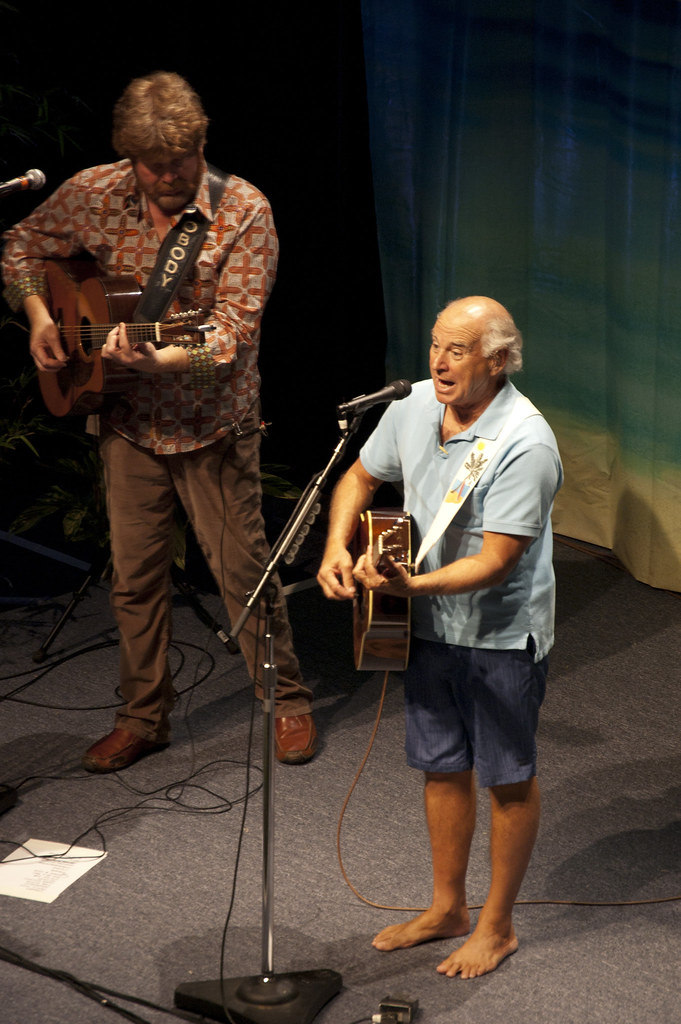In this indoor concert setting, the stage is carpeted and predominantly features shades of gray. Toward the top right of the image, a multi-colored curtain forms the backdrop. Center stage, two men stand at microphones, each strumming an acoustic guitar hooked up to electric jacks. 

The man on the left is a large, middle-aged, bearded white man with thick, brown hair parted in the middle. He wears brown pants, brown shoes, and a brown-orange shirt adorned with a repeating cross pattern. His guitar is strapped with a black band, and various cords surround him.

To his right stands an older, barefoot man in his 60s, balding with gray hair on the sides. He dons jean shorts and a blue polo shirt and strums his guitar using a white strap adorned with designs. With his mouth open, he appears to be singing. Both musicians are illuminated under stage lights, highlighting an array of colors, including gray, black, brown, red, light blue, green, and yellow, while they bring their performance to life.